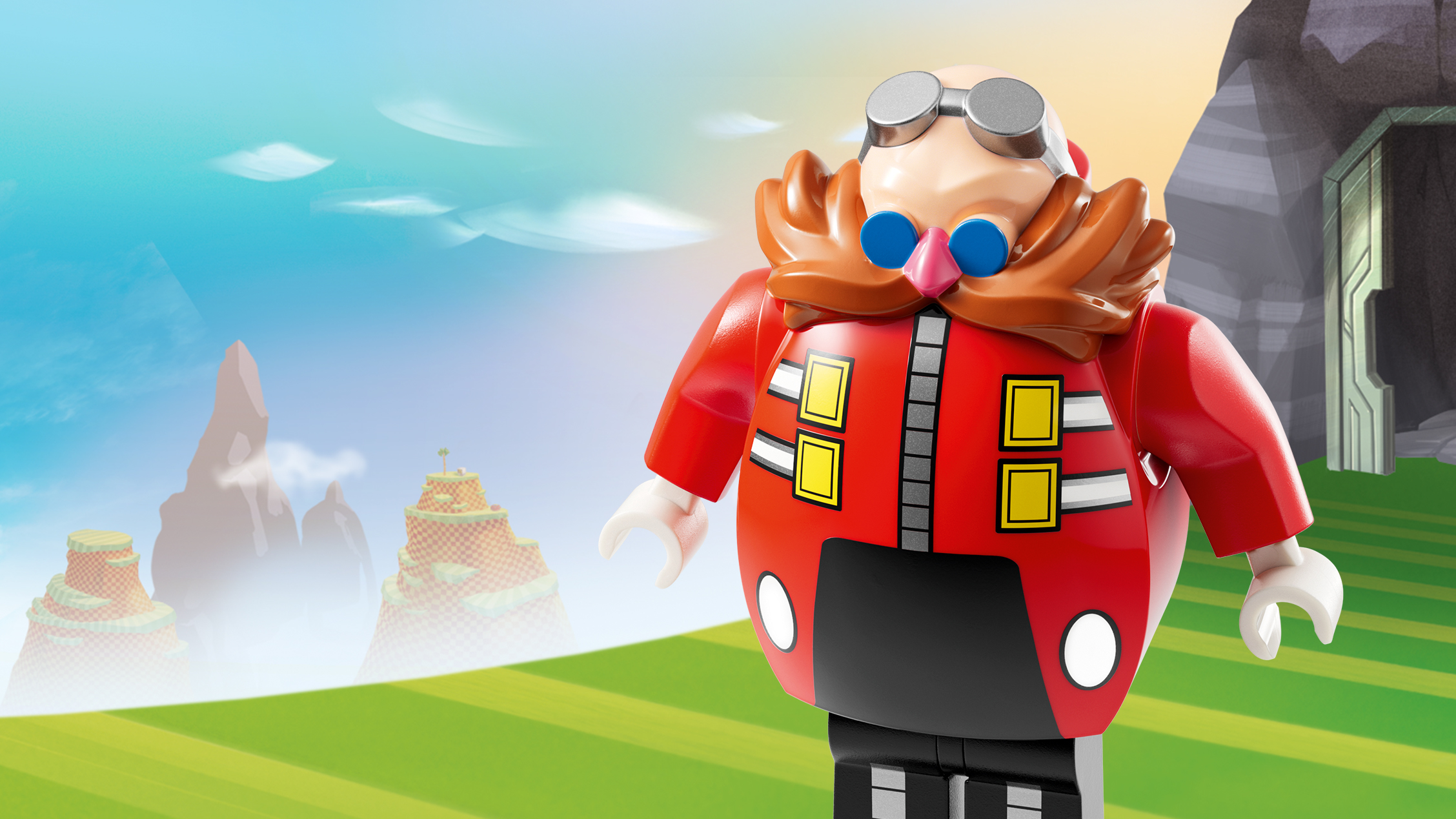The image is a computer-generated depiction of Dr. Eggman from Sonic the Hedgehog, rendered as a Lego figure. Dr. Eggman has a distinctive bald, white head adorned with silver goggles on top and blue glasses over his blue eyes. He sports a massive auburn mustache that extends well beyond his face, and his nose is prominently large and pink. His outfit consists of a red jacket, reminiscent of a fireman's jacket with yellow squares and various silver clasps and red buttons, as well as two white buttons near the bottom. He wears white gloves and black pants. The backdrop is a rocky cave with green doors flanked by brown and gray mountains with patches of grass. The character stands on striped green terrain under a cyan sky with clouds.